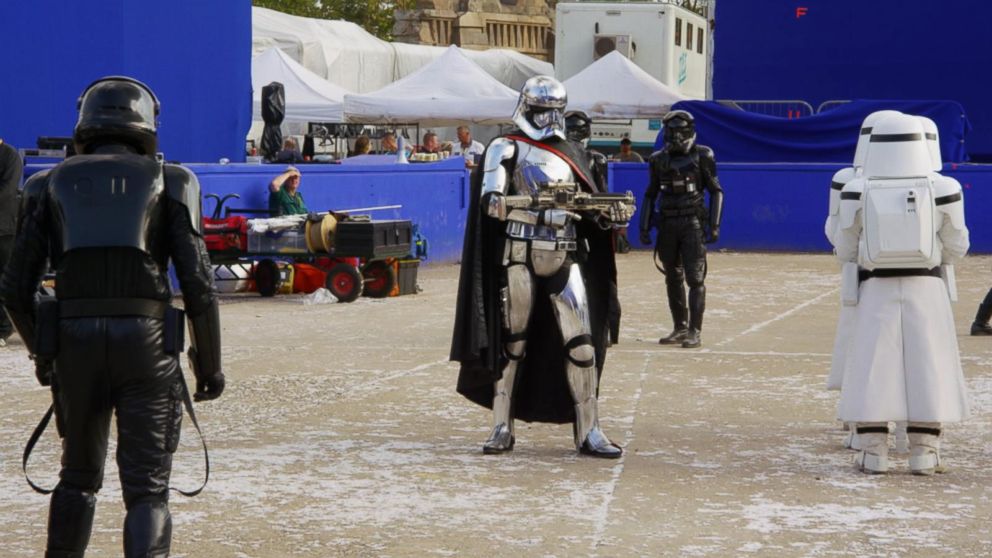This image captures a detailed scene that appears to be from a Star Wars-themed event, perhaps a convention or a movie set. The photo depicts an outdoor arrangement, possibly on a snowy or grey field, with a blue stage set up beyond the main action. White tents and walls frame the background, suggesting a larger setup.

In the center of the image stands a character in silver armor with a matching helmet, holding a gun and adorned with a black cape. Surrounding him are various Star Wars characters in uniform: to his right is a figure in white armor, possibly a stormtrooper, with detailed gear including a white helmet and backpack; to his left is a character in black armor, reminiscent of Darth Vader, though only the back is visible. Another figure in black armor is located in the left-hand corner, showing a close-up of the uniform.

In front of the stage, red and black equipment is visible, adding a sense of realism or functionality to the scene. A person in a green shirt, sitting and shading their eyes with their hand, is present near this equipment, watching the activities unfold.

The setting appears to be captured in daytime, with a blue backdrop that might be part of set dressing or blocking out other structures. No text or signage is visible, adding to the immersive Star Wars ambiance of the scene. The attention to costume detail and the spread of characters across the scene contribute to a rich, organized depiction of the themed event.